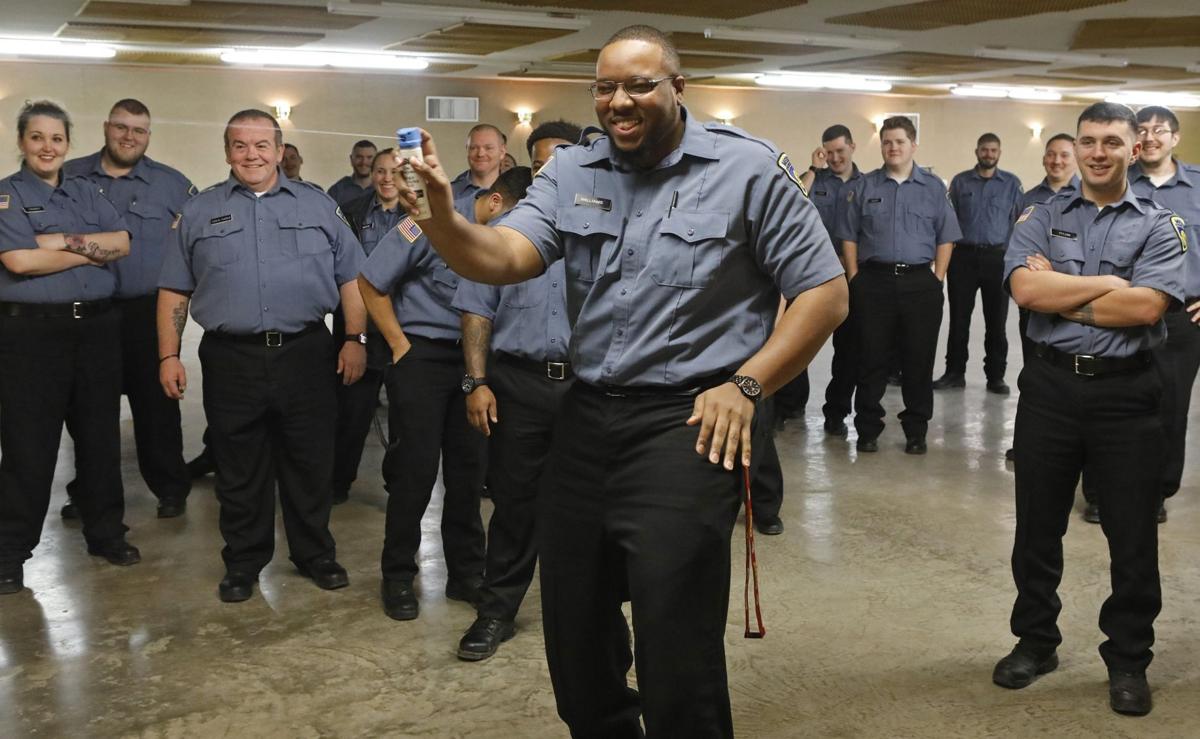In this horizontally oriented, realistic photograph taken inside a large beige and white building, possibly a basement, parking garage, or convention center, about 20 individuals, presumably security guards or police officers, stand attentively. They wear matching uniforms of black pants and blue shirts adorned with patches. The room features a beige floor and walls, a white and beige ceiling with overhead lighting, and additional lights on the back wall.

The focus is on an African American man at the center of the scene. He has short black hair and wears glasses, a black watch, and a brown string hanging from the left side of his belt. In his right hand, he holds a can with a white cylinder and a blue top, from which he appears to be spraying some substance, possibly pepper spray, towards the left of the camera. Despite the serious context, he is smiling. His actions and appearance create a striking focal point amidst the surrounding group, who are similarly uniformed and mostly composed of individuals in their twenties to forties.